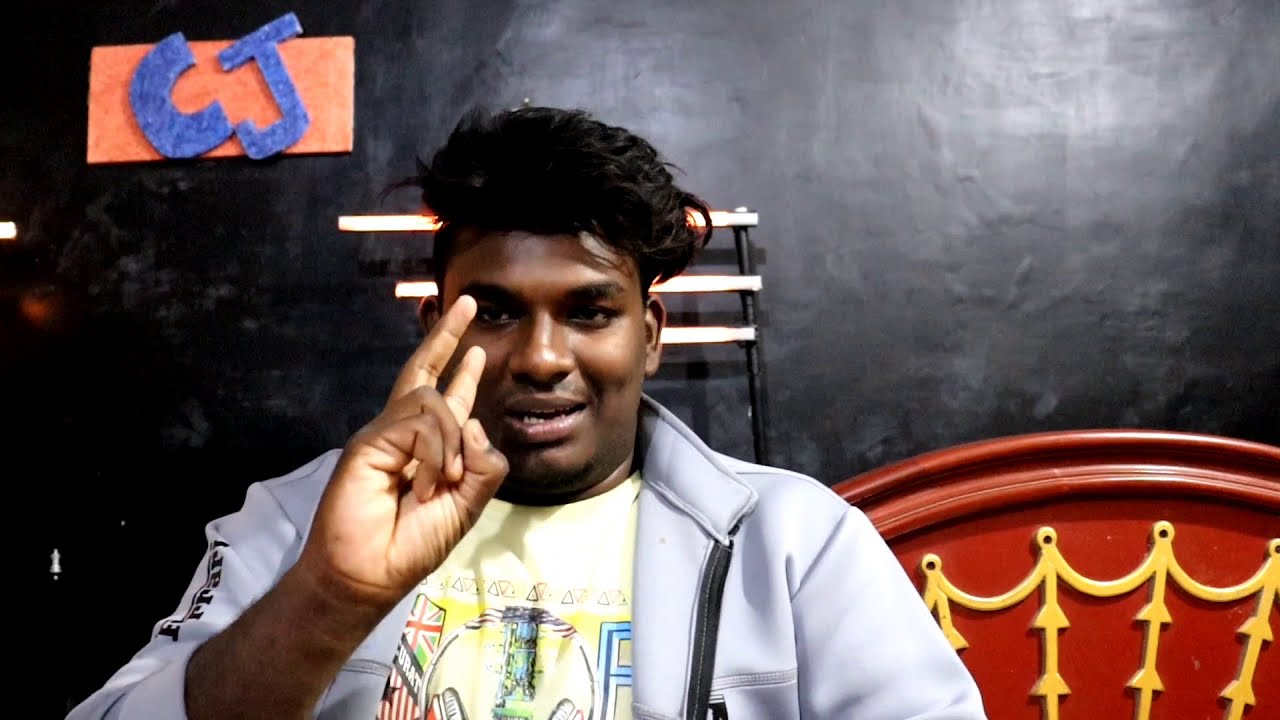The image depicts a young African American man in his twenties, seated indoors against a dull black wall that reflects light. The man has dark skin and short, fluffy black hair. He wears a white or light gray jacket over a white t-shirt that bears the flag of Great Britain on the left side. He is holding up his right hand with his middle and ring fingers extended. He appears to be in mid-conversation. In the background to his right, there is a red headboard or ornamental object with gold designs. On the top left corner of the image, a peach-colored rectangle with the blue letters 'CJ' is visible. A black structure with gray or illuminated lines is directly behind his head, completing the scene.